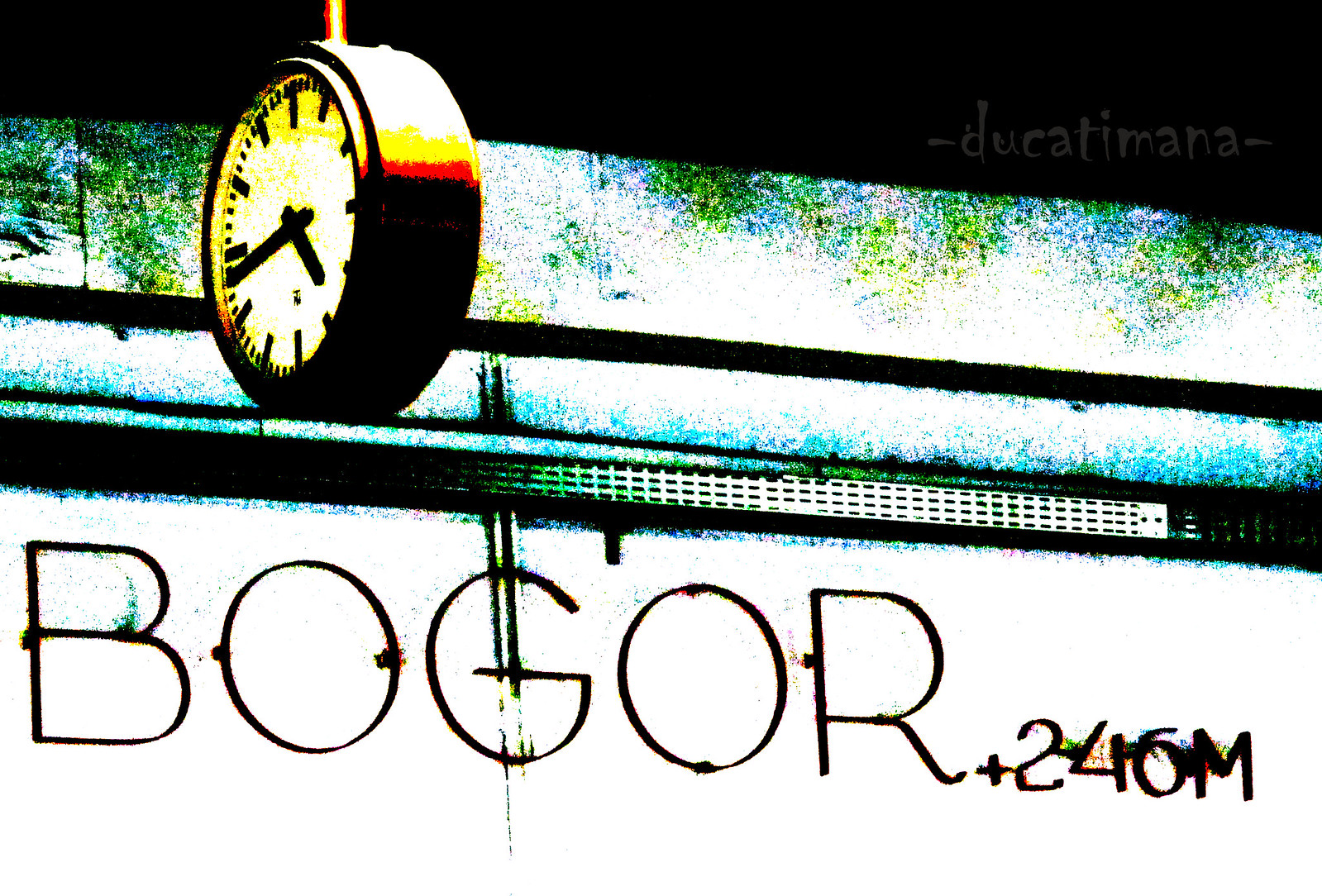This heavily distorted image depicts an exterior view of a building, primarily with a white wall. The top section features a notable black area, leading into a rectangular band with a mix of bluish, greenish, and yellow tones. In the top left corner, a clock is prominently displayed; it has a partially gold, partially black rim and a face that is white with black hands, showing a time close to 5:45. The clock face lacks traditional numbers, using slashes instead. In the top right corner of the image, there's a watermark that reads "Duke of Tamanna." The bottom section of the image displays text that appears as "BOGOR," followed by "+246M." The image is heavily distorted with several artifacts and improper color balancing, contributing to its abstract, artwork-like appearance.